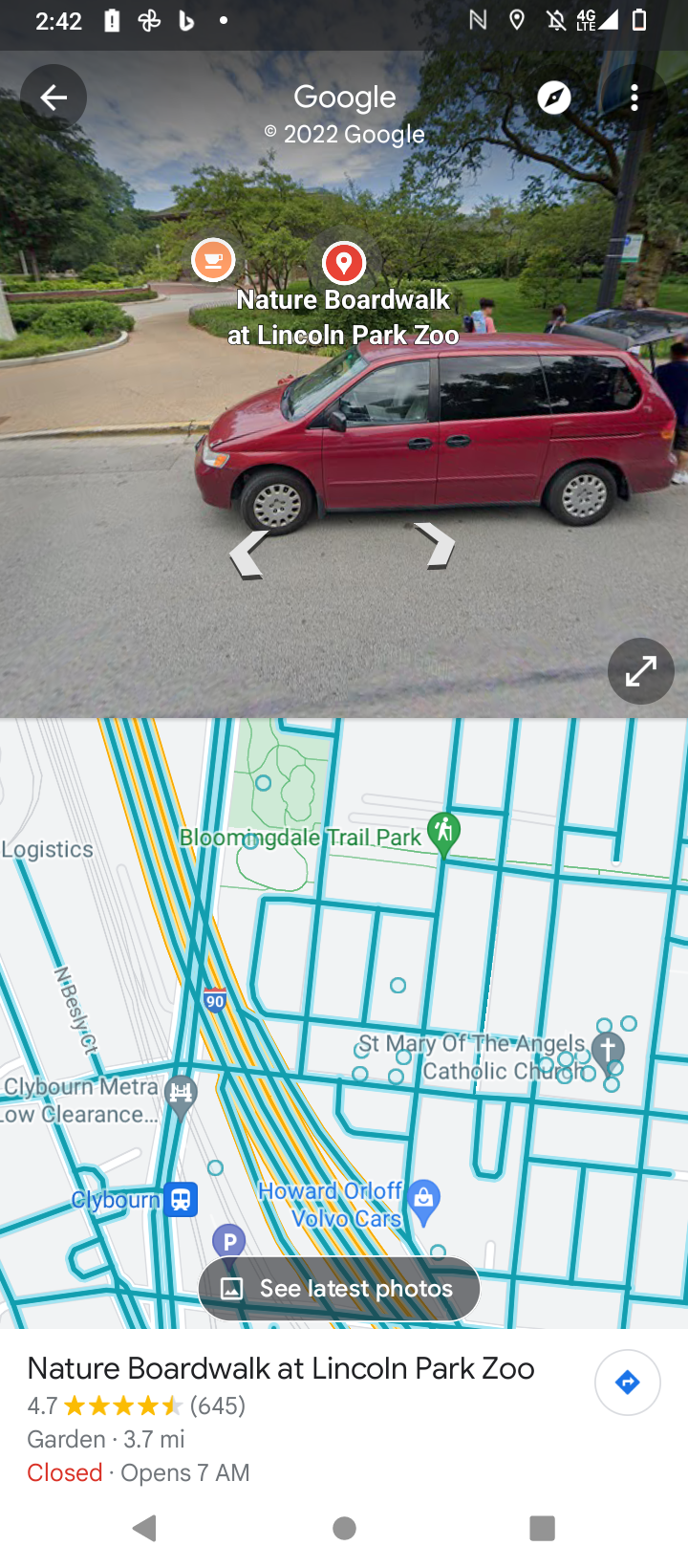A mobile screenshot displays a Google Maps interface. At the very top, a black strip shows the time, 2:42, along with a "Google 2022 Google" label. Below this, in the middle of the upper section, text reads "Nature Boardwalk at Lincoln Park Zoo." 

Foregrounded in the image is a cranberry-colored minivan facing left on a gray concrete road. Behind the vehicle, a curved concrete sidewalk meanders through a park-like setting, bordered by grass and dotted with trees. 

The lower half of the screenshot presents a map interface. At the bottom, a label indicates "Nature Boardwalk at Lincoln Park Zoo," boasting a 4.7-star rating from 645 users. Additional information reveals that the garden is 3.7 miles away and currently closed, with an opening time of 7:00 AM marked in red letters.

Further details on the map include labels for various locations, one of which is the "St. Mary of the Angels Catholic Church." Blue lines highlight different routes and areas of interest, though some text remains difficult to read.